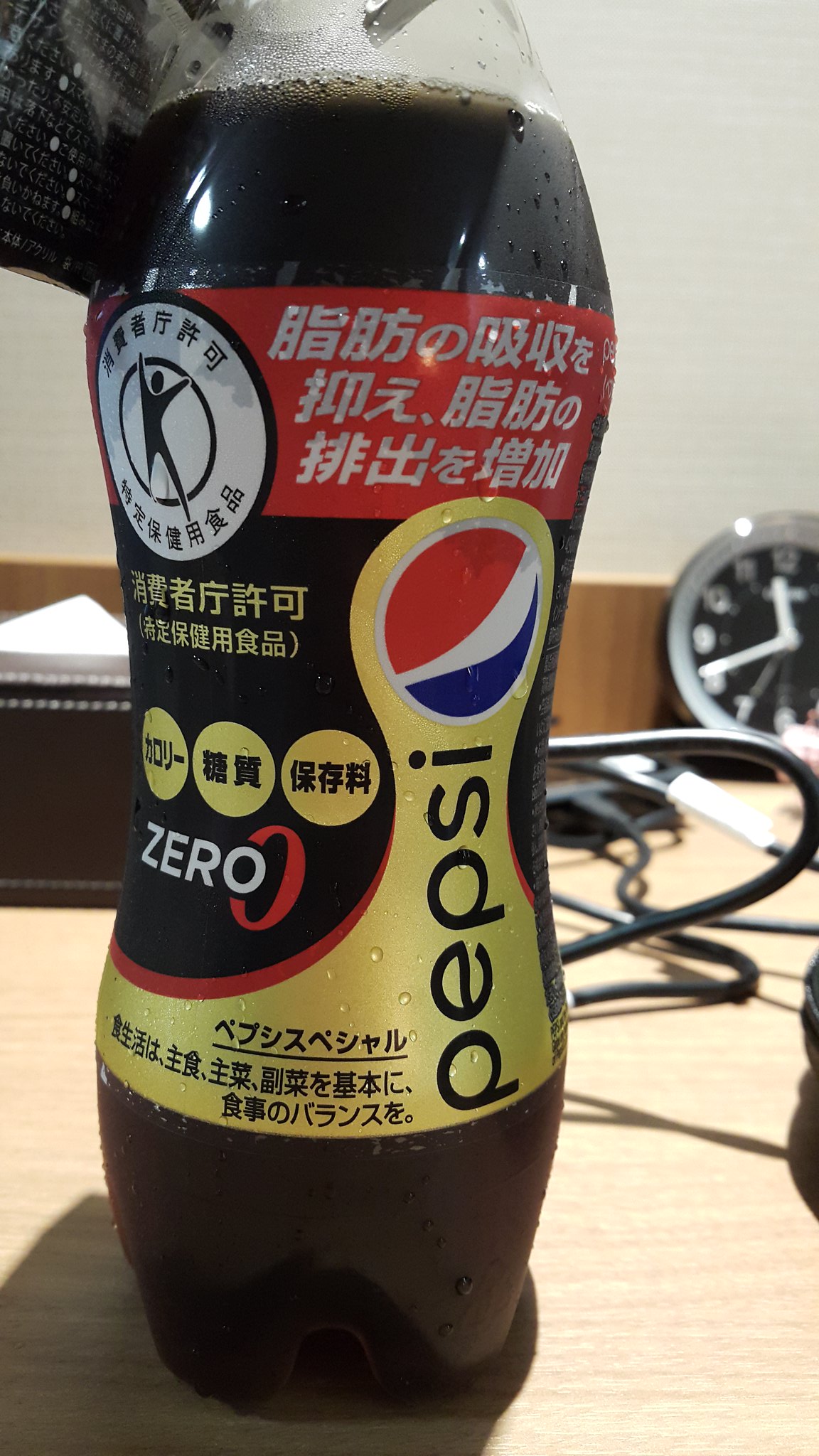A photograph captures a plastic Pepsi bottle positioned towards the lower left, showcasing both the front and the right side of the bottle. The bottle, unopened and missing its cap in the frame, rests on a wooden desk. The bottle's label features Japanese or Chinese writing, with the iconic Pepsi logo—a red, white, and blue circle—prominently displayed on the side, oriented vertically. In the background, a section of a leather binder and a round desk clock are partially visible, adding context to the setting.